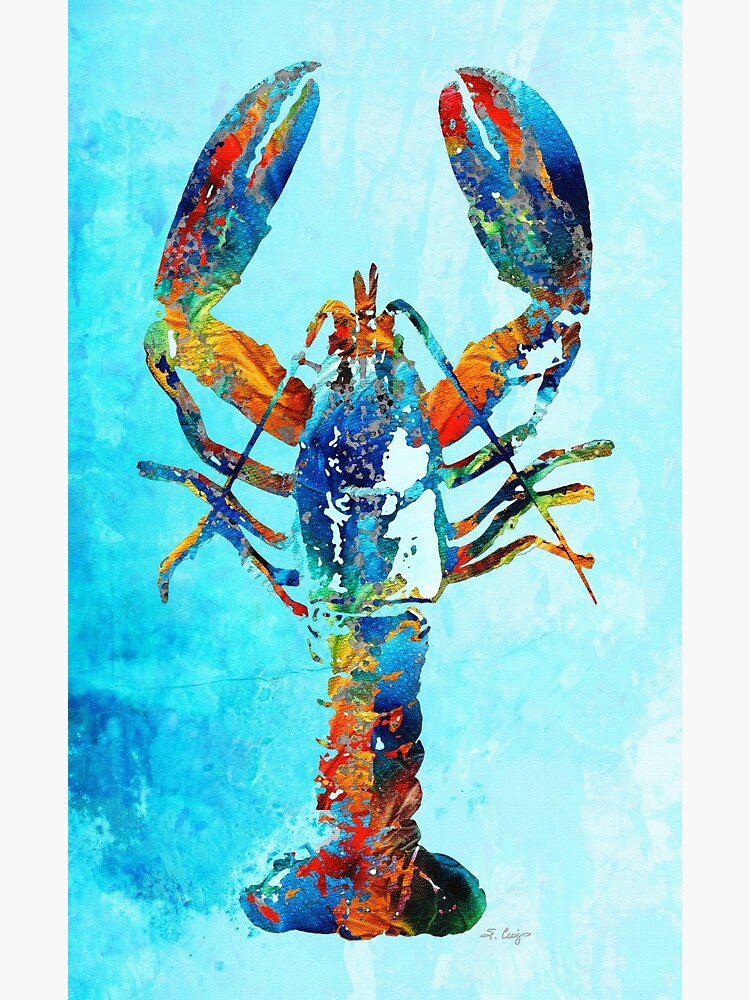This image features a painting of a lobster rendered in an abstract, sponge press style that results in an inconsistent, yet compelling border. The lobster, viewed from a top-down perspective and facing upwards, is a striking array of colors ranging from deep blue at its core to gradients of red, yellow, green, and lighter blue. Its claws are splayed outwards, and its feelers angle back towards its body. The backdrop is a pastel blue that exhibits splotchy variations in hue, with a darker blue patch in the bottom left that suggests the impression of water. In the bottom right corner, there's a small gray cursive signature by the artist, marked S. Kujo. The overall composition combines vivid, heat map-like color transitions with a soft, non-realistic form.